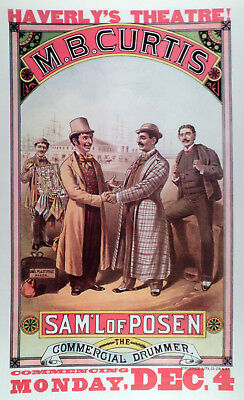This image is a detailed, old-school poster, likely from the late 1800s to early 1900s, advertising a performance at Haverly's Theatre. The backdrop of the poster is a light blue sheet of paper with an ornate pink border and black circular details in each corner, adorned with an unclear pattern.

At the top, in hand-drawn red text resembling felt-tip, the poster announces "Haverly's Theatre!". Below this, in an arching black text on a pink background, it states "M.B. Curtis". The central imagery features four Caucasian men dressed in period attire. 

The two men in the foreground are engaged in a handshake, leaning towards each other in long overcoats extending to their ankles. The man on the left wears a checkered coat, brown three-piece suit, and a bowler hat, along with a black mustache. The man on the right sports a brown coat, red three-piece suit, a top hat, and similar facial hair. Behind them, to the left, stands another man dressed in a brown coat and dark trousers, holding a suitcase or briefcase with scarves or neckties dangling from it, suggesting he might be a vendor. The fourth man, positioned to the right, is in a gray suit and short jacket, leaning against a wall with one leg bent, wearing glasses and sporting short, curly hair parted in the middle.

Text at the bottom of the poster reads "Sam'l of Posen, The Commercial Drummer," followed by "Monday, Dec 4" in red letters. This elaborate poster vividly captures the essence of an advertised theatre performance, blending intricate details with historical elements.